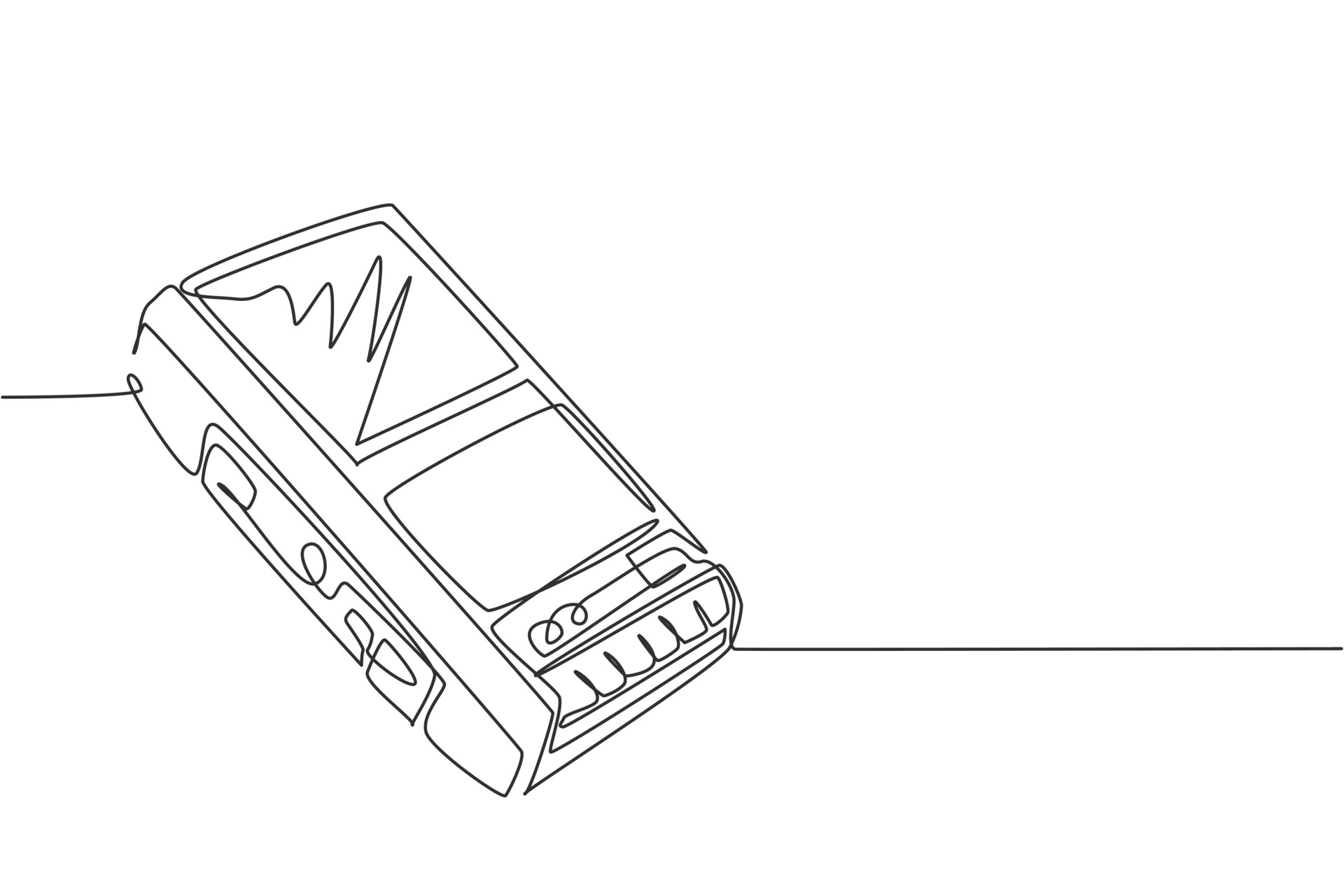This is a black and white line drawing of an old-fashioned cassette recorder, done in a continuous pen stroke with no line breaks. The line starts from the left, looping back and forth to form the entire outline of the recorder. The drawing details a central section for the cassette tape, flanked by large, pressable buttons on the side for functions such as stop, play, and record. The simplistic yet detailed design allows one to trace the entire image from start to finish in a single, uninterrupted line.